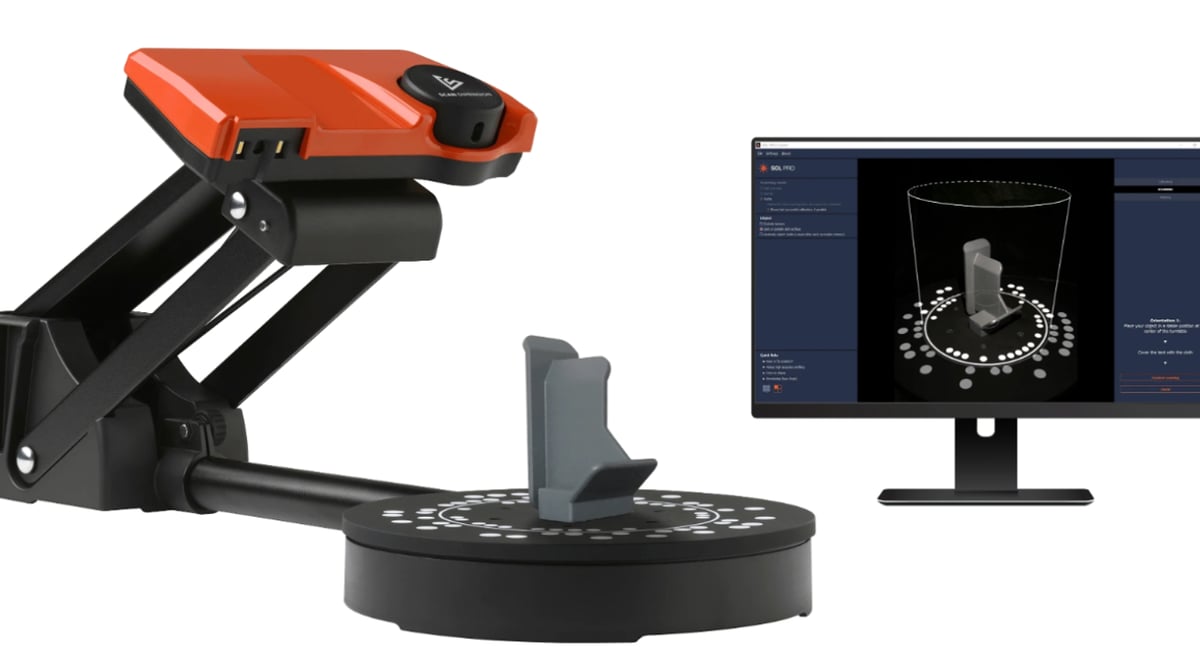The image depicts a sophisticated setup involving imaging and computing equipment. On the left side, there is a device that appears to be some sort of camera or projector mounted on a robust, black metal stand designed for stability. The device showcases an orange top, contrasted by the black components of the stand, including a small arm extending at an angle that holds a circular piece. This circular component features a gray clip, presumably for securing objects. Additionally, a black circular pad at the base is adorned with numerous white dots.

On the right side of the image, a computer monitor displays a detailed view of a clear cylinder positioned over the gray clip and circular section of the base seen on the left. The monitor itself has a black frame and a base, and its screen has blue sections flanking a central black area where the detailed image of the cylinder and gray clip is projected. The alignment of the white dots on the black pad with the display on the monitor suggests that this setup is used for precise 3D or computer imaging. The entire scene is set against a pure white backdrop, enhancing the visibility of the described elements.